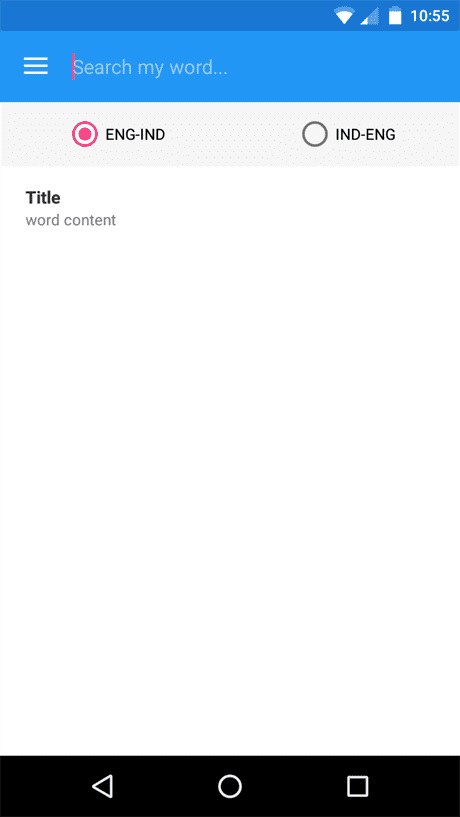Here is a cleaned-up and detailed descriptive caption for the image:

---

The image is a screenshot taken from a cell phone display. At the very top, there is a search bar labeled “Search my word” inside a royal blue rectangle containing three white horizontal lines on the left. Adjacent to the search text, a red cursor is visible, followed by an ellipsis. Below this, there is a form with two distinct sections labeled "ENG-IND" and "IND-ENG." The "ENG-IND" option is marked with a solid red circle, indicating it is selected, while the "IND-ENG" option, to the right, is outlined by a gray circle showing it is unselected.

Further down the screen, a title label appears in bold black text, beneath which a subtitle reads “word content” in gray font. The rest of the screen background under these labels is plain white, leading to a solid black bar spanning the bottom width of the display. This bar has three symbols: a white triangle pointing left, a white circle, and a white square, each spaced apart sequentially.

In the upper right corner of the screen, the status bar shows the time as 10:55, and icons for battery life, Wi-Fi connection, and another signal indicator shaped like a triangle.

---